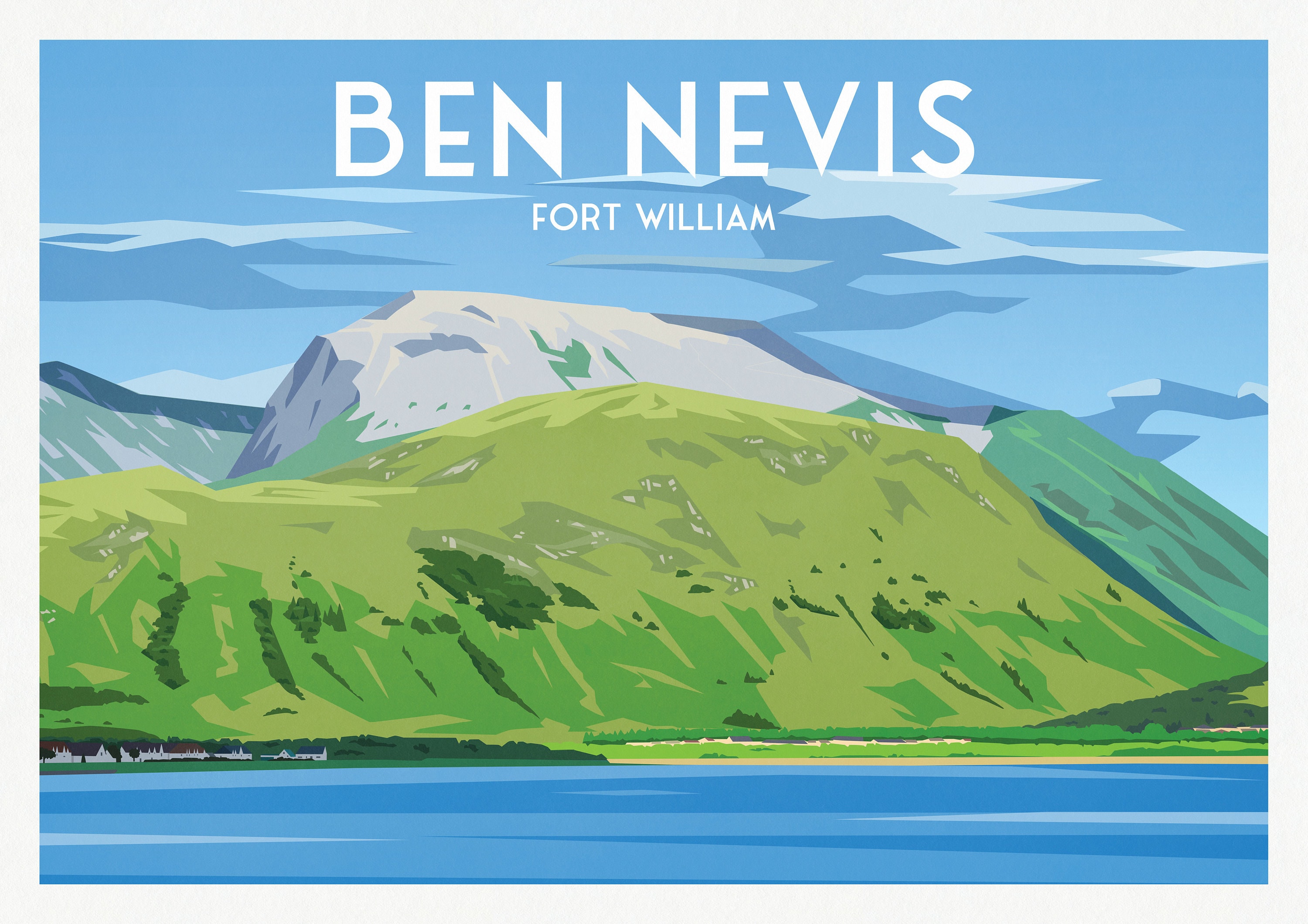This is a detailed digital painting of a tranquil lakeside scene dominated by a picturesque, grassy hill and a towering mountain in the background. The serene lake, depicted in a deep dark blue, stretches across the foreground, with several small houses nestled along its bottom edge, especially concentrated in the lower left corner. The central grassy hill is rendered in various shades of light green, complemented by patches of gray and darker green brush. Rising majestically behind is a larger mountain in light gray, snow-dappled at its peak, suggesting the presence of rugged rock slides. Above, a pale blue sky sets the scene, adorned with a couple of geometric, impressionist clouds. At the top center of the painting, the words "Ben Nevis" are prominently displayed in white, with "Fort William" written in a smaller white font directly below. This meticulous digital artwork effectively captures the natural beauty of the landscape through its impressionistic style and vibrant, contrasting colors.